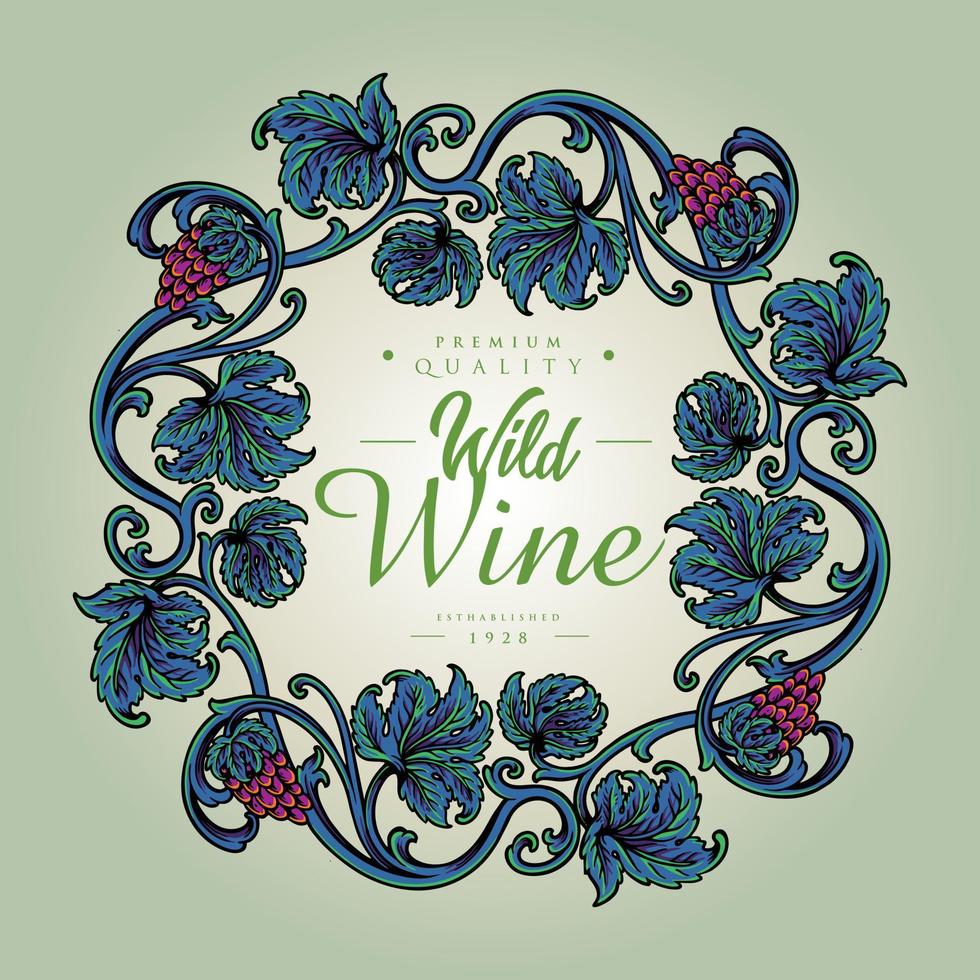The image is square-shaped with a light grayish-green background that transitions to white at the center. At the heart of the design is a circular grapevine rendered in blue and green hues, adorned with exaggerated leaves and clusters of red and purple grapes. There are four equidistant bunches of grapes around the vine. The central text is in a sage green color: at the top, in smaller letters, it reads "Premium Quality" with a dot on either side; below, in a larger cursive font, it states "Wild Wine"; and at the bottom, in smaller letters again, it notes "Established 1928."